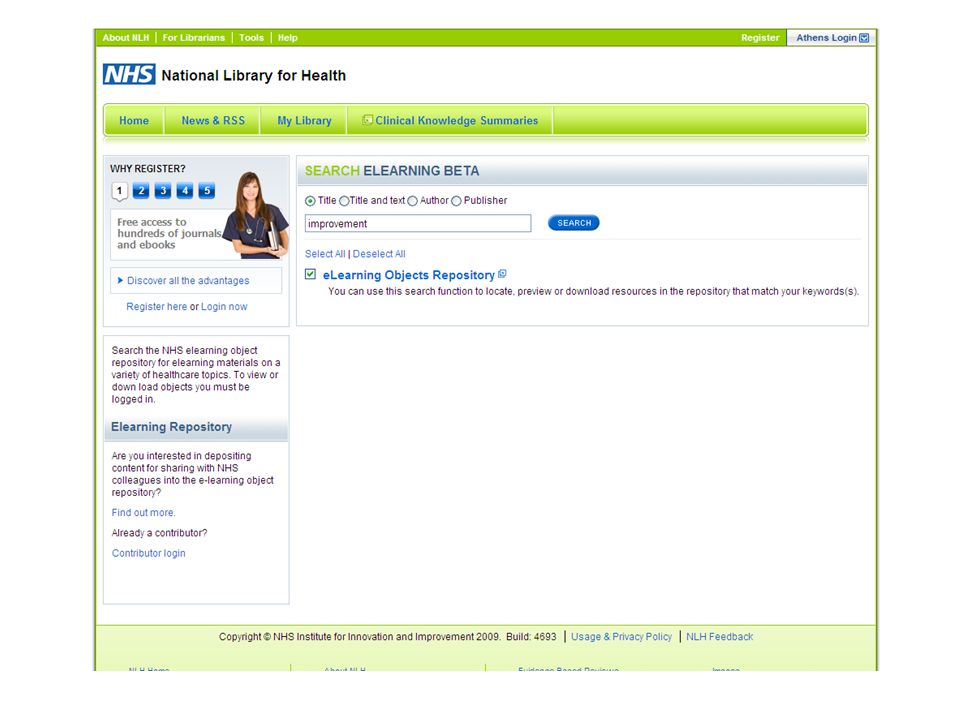The image showcases a vibrant digital interface for the National Library for Health's (NLH) Leprelain Tooth Help portal. The overall layout is set against a structured green box. 

At the top left corner, tabs are labeled 'NLH' for Leprelain Tooth Help, while the top right features navigation options: 'Register,' 'Attends,' and 'Login.' Directly below these on the left side is the 'NHS' tab, standing out with its white text against a blue background. Adjacent to this, in a descriptive blue text, is the title 'National Library for Health.'

Beneath this primary section lies an array of green-background tabs with blue text. The tabs include 'Home,' 'News,' and 'RSS,' followed by 'My Library' and 'Clinical Knowledge Summaries.' Below, a section titled 'Why Register' details five progressive steps, with the first step highlighted in white to indicate it's being displayed. This step explains the benefits of free access to hundreds of journals and e-books, encouraging users to explore all advantages and provides 'register here' or 'log in now' options.

At the bottom of the image, a section guides users on searching the NHS e-learning objects repository. It highlights the need to log in to view or download e-learning materials on various healthcare topics and invites contributors to log in and share content with NHS colleagues. 

On the right side, a search interface is visible. It features a beta search for e-learning resources, categorized by title, title and text, author, and publisher. The blue search box displays 'Improvement' as a sample search query. The search results, labeled 'e-learning objects repository,' detail how users can utilize the search function to locate, preview, or download resources matching their keywords.